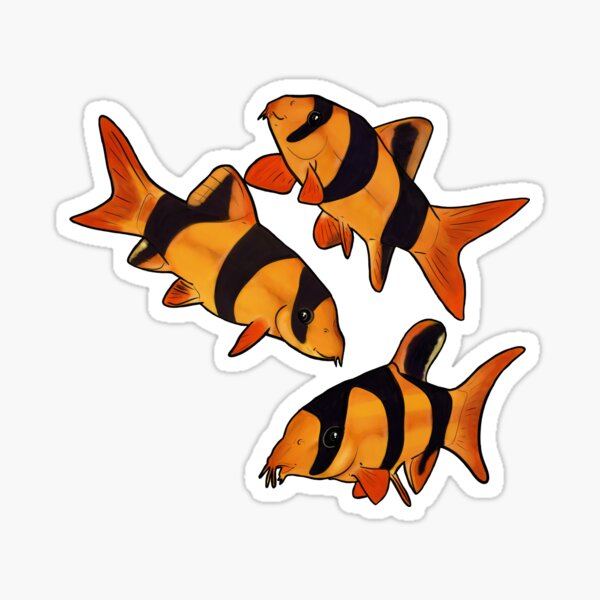The image features a sticker of three cartoon-style koi fish set against a bright white background, which itself is bordered by a light gray background. The koi, each adorned with wide vertical black stripes, are depicted in vibrant golden hues with red highlights at the edges of their large fins, particularly towards the back. Each fish has distinctive tendrils or whiskers near their mouths, helping to identify them as koi rather than goldfish. The fish have small beady black eyes and are arranged vertically, though not all face the same direction. The white background serves as a cutout that encircles all three koi, making the bright colors and intricate details stand out vividly against the light gray border.